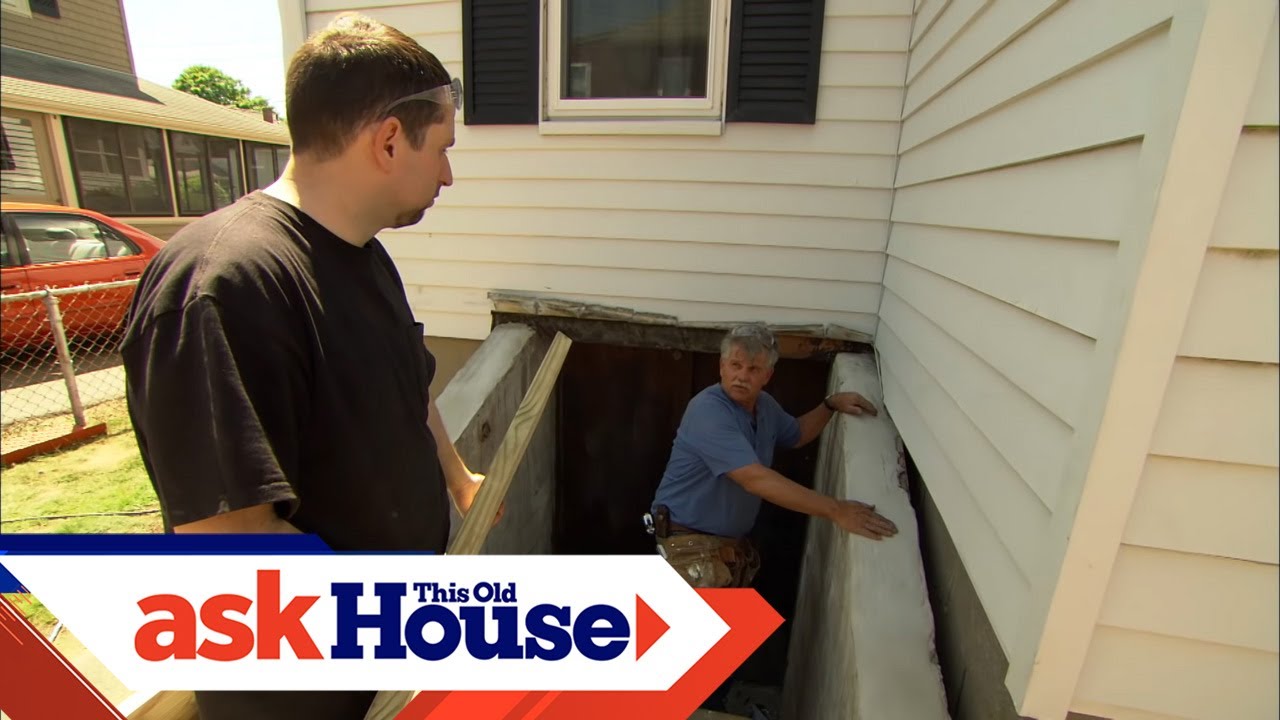In the image, two men are standing outside a vintage, off-white clapboard house with green shutters. The older man, who has gray hair, wears a blue t-shirt and is positioned at the bottom of a stairwell that appears to lead into the cellar of the house. The slightly younger man with dark brown hair and a black t-shirt stands at the top of the basement entrance, engaging in conversation with the older man. This scene seems to capture a moment from a house restoration project, part of the "Ask This Old House" series, as indicated by a banner at the bottom left of the image. The banner features the text "Ask This Old House," with "Ask" in red and "This Old House" in blue, set on a white background. The house next door on the left has a red car parked in the driveway. The entire setting suggests the two men are likely discussing the foundation or a related issue of the house they are working on.